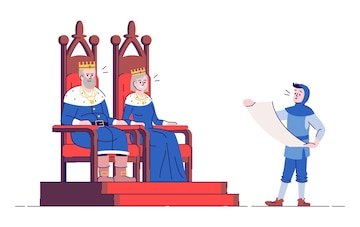In this vivid cartoon illustration, a king and queen from the Middle Ages are seated on a two-step wooden platform, adorned with red steps and high-backed chairs with red seat cushions. Both royalty are dressed in resplendent blue and white outfits, accessorized with golden crowns and medallion necklaces. The king, with his short gray hair, gray beard, and tan boots, contrasts with the queen, who wears a blue dress and has short gray hair styled in a page boy cut. They share a serious expression as they listen to a royal emissary standing before them. This figure, possibly a servant or herald, is also dressed in blue with knee socks, brown shoes, and a blue collar that reveals the top of his brown hair. He is reading aloud from an unrolled white scroll, with lines drawn near each character's head to indicate that they are engaged in a dialogue.